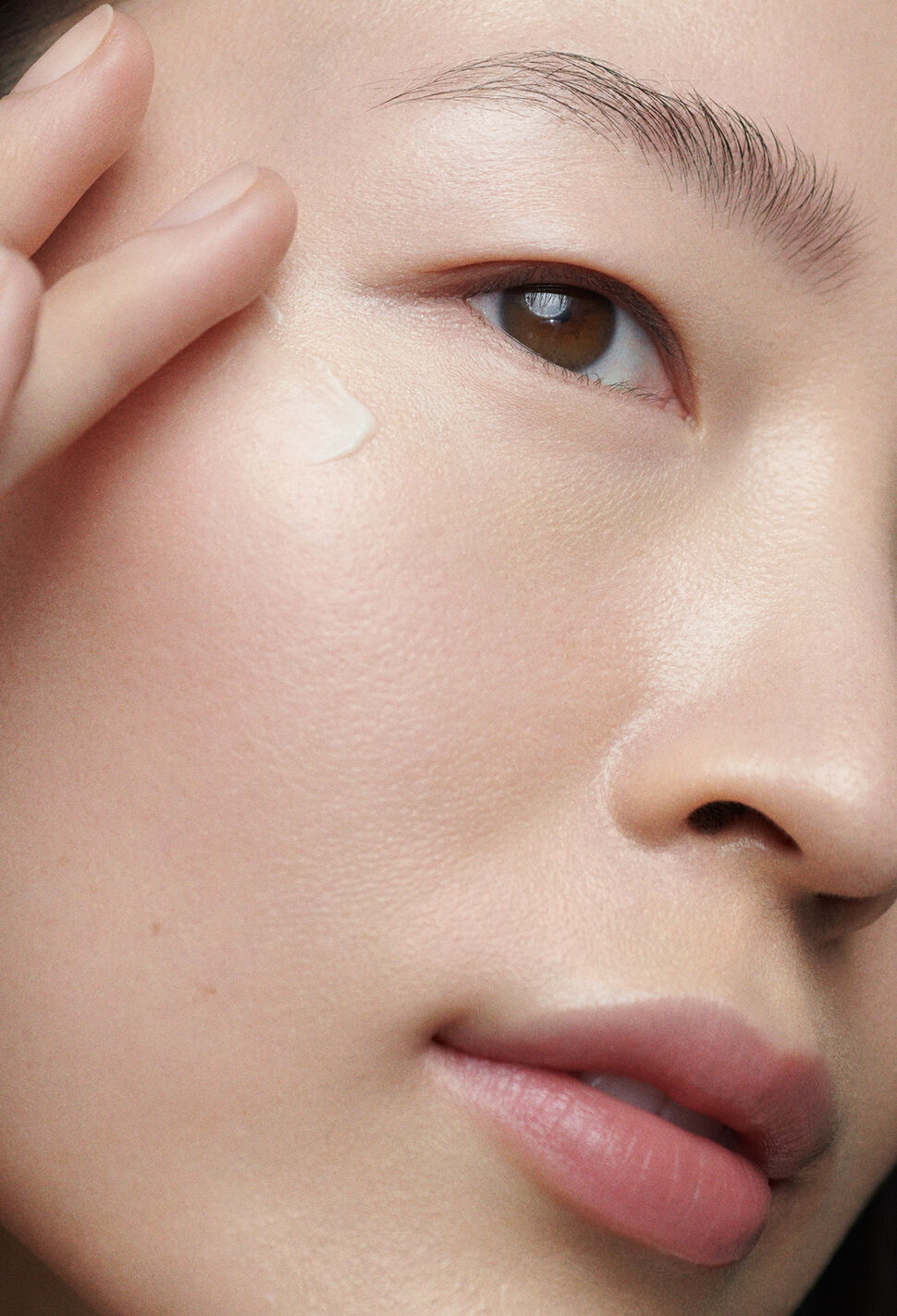This image features a close-up of an Asian woman with exceptionally clear, smooth skin that is very fair in color. Her single visible eye is brown, framed by perfectly shaped darker eyebrows, while her eyelashes and the finer textures of her skin are clearly visible, indicating minimal to no makeup. The woman's sultry, naturally pink lips are partially open as she appears to be applying a white cream, likely a lotion or serum, to her cheek just below her eye. The light reflecting in her eye and the shadow of her hand against her face add depth and realism to the photograph, suggesting she might be looking into a mirror. Her nose is positioned along the right side of the image, with her fingertips appearing at the top left, gently rubbing the product into her skin. The image, potentially edited to enhance smoothness, presents a highly detailed and intimate view of her features, with a hint of rosiness on her cheeks and a slight opening of her mouth.